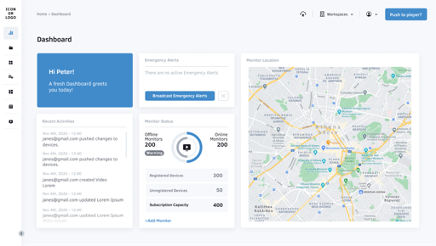This image depicts a computer webpage, specifically a dashboard interface. On the left-hand side, a navigation panel labeled "Dashboard" is visible, though it appears quite small. The images across the dashboard are similarly small in size, contributing to a compact design.

In the upper-right corner, there is a clickable blue box, distinct against the interface's background. Dominating the upper section is a prominent blue box displaying a greeting, “Hi Peter!” in white text, followed by additional white text underneath, though the content of these words is not specified.

Below this greeting section, a white column extends downwards, containing various elements. In the second row of this column, there is another white box featuring a smaller blue box within it. This section mentions "offline" and "online" statuses, each associated with the number 200.

Additionally, an image of a circle is displayed, divided into a blue segment on the right and a gray segment on the left, possibly representing some form of data segmentation.

To the right of these elements is a detailed map. The map showcases a network of gold lines indicating main roads, while white lines denote other roads, adding to the geographical depth of the interface. This detailed and organized arrangement of elements suggests an analytical or monitoring application for the dashboard.